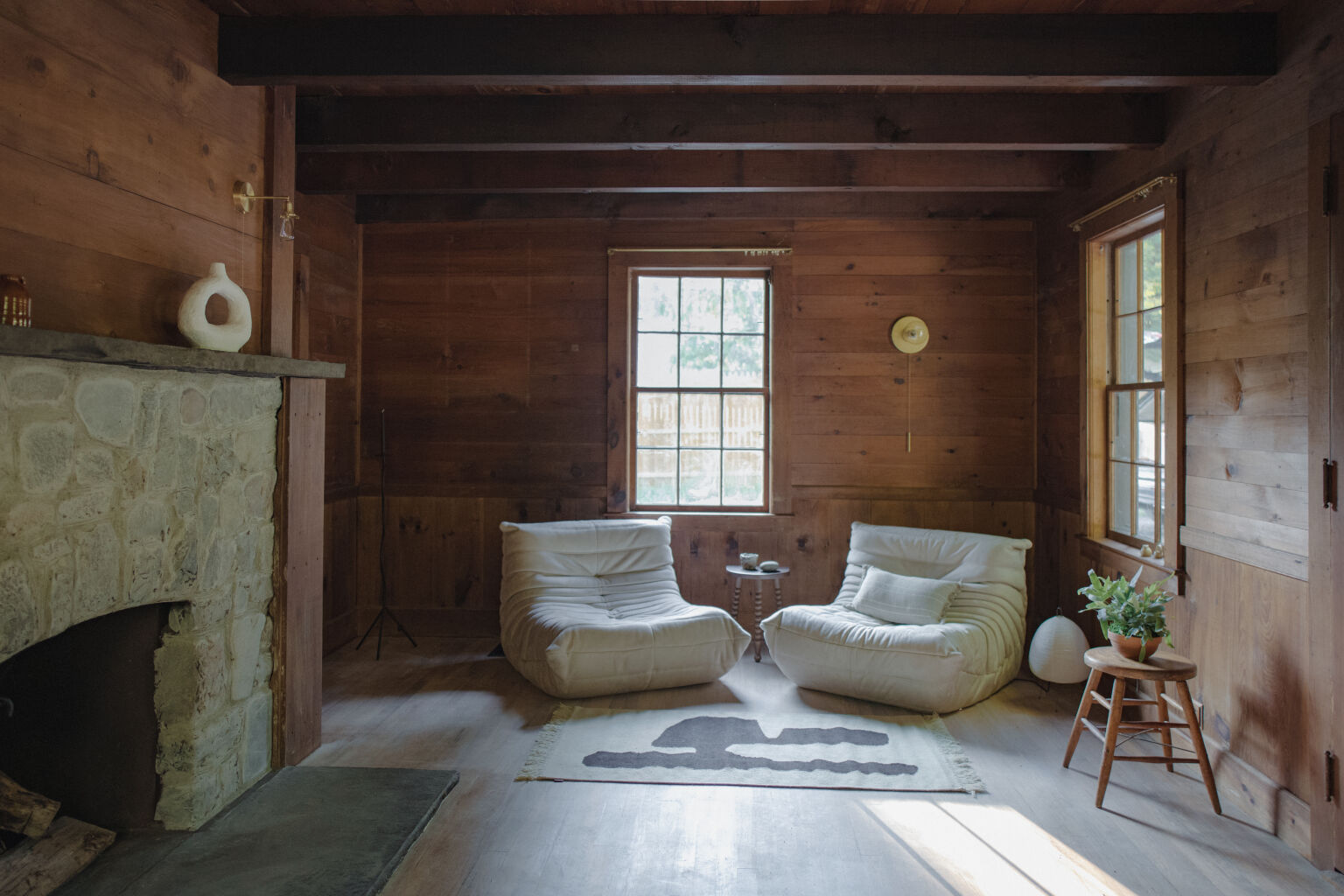The photograph captures the cozy, sunlit interior of a rustic wood cabin. The room is bathed in dappled natural light, highlighting the rich textures and warm tones of the space. The walls are finished with broad, flat planks in a shiplap style, creating a seamless wooden embrace that climbs up to the ceiling, which features stout, darker wooden beams. The floor is also wooden, composed of wide, polished planks.

Dominating the left side of the image is a stone fireplace with a hearth that looks like slate. Peeking out from the fireplace is a log, though no fire is currently burning. Above the rustic wooden mantle, which supports a white donut-shaped pottery vase, hangs a brass sconce. This historical touch adds to the cabin's quaint charm. 

The room's focal point is further enriched by the seating area set before a large, sun-drenched window at the back. Two cushiony, off-white, armless chairs lie directly on the wide plank floor, resembling partially folded futons. They cradle a small bistro-style end table. The chairs rest upon a small, fringed area rug, tying the seating arrangement together in comfort. Another window on the right side of the room frames radiant beams of sunlight, illuminating a round wooden stool that supports a potted plant.

Overall, the photograph exudes warmth and tranquility, showcasing the rustic elegance and inviting simplicity of cabin life.